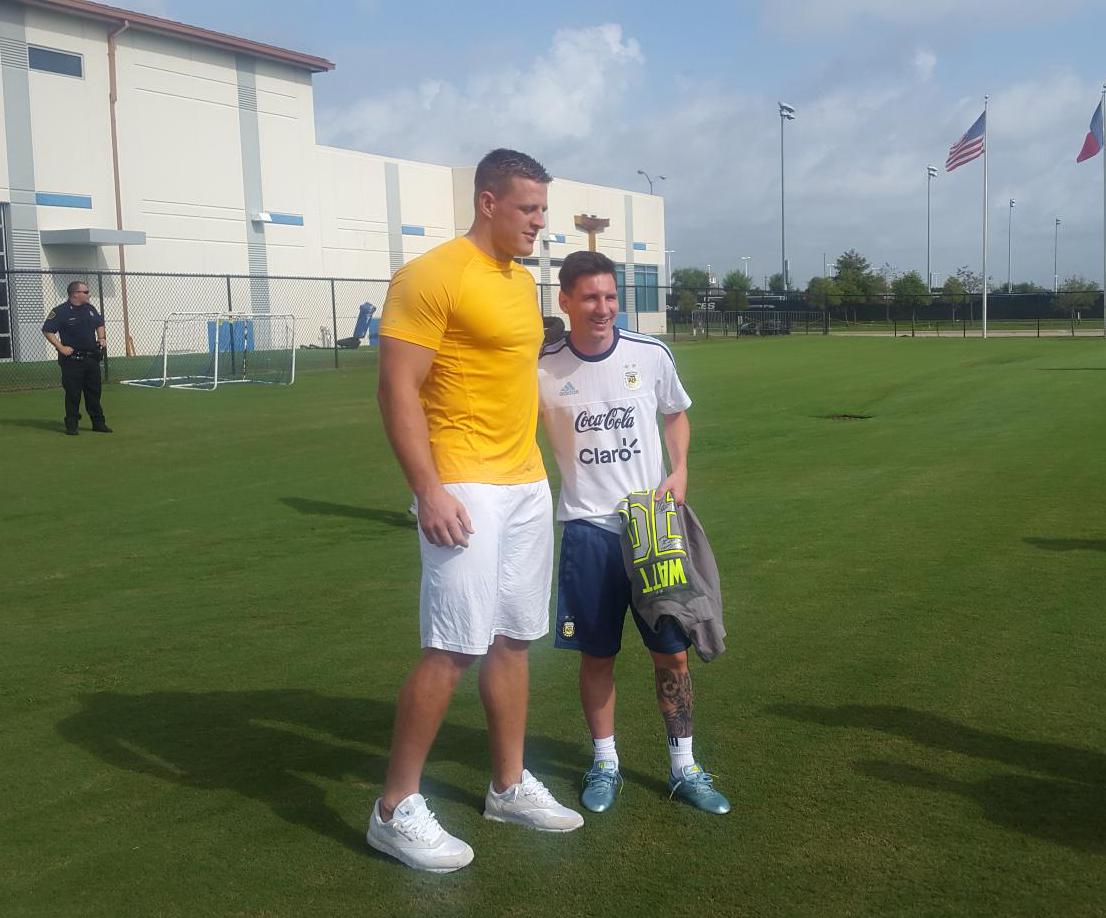The scene is an outdoor sports field on a partly cloudy day, with patches of blue sky visible amidst fluffy clouds of varying shades of white and gray. In the background, different types of stadium lighting structures rise above a row of trees, alongside which the American flag and part of the Texas flag wave in the wind. A multi-story white building stands in the distance.

On the green grass field, a police officer is present, looking to the right of the viewer's perspective. Near the officer, there is a soccer goal, and center stage are two prominent figures: JJ Watt and another individual, likely a soccer player. JJ Watt is dressed in white shorts, white tennis shoes, and a yellow top, while the soccer player sports an Adidas soccer jersey emblazoned with the Coca-Cola sponsor logo, blue shorts, white socks, and blue shoes, along with a visible leg tattoo. 

The soccer player holds a signed JJ Watt jersey in one hand while his other arm is draped around JJ Watt's shoulders. Both are smiling for a picture, capturing a moment of camaraderie on the field.